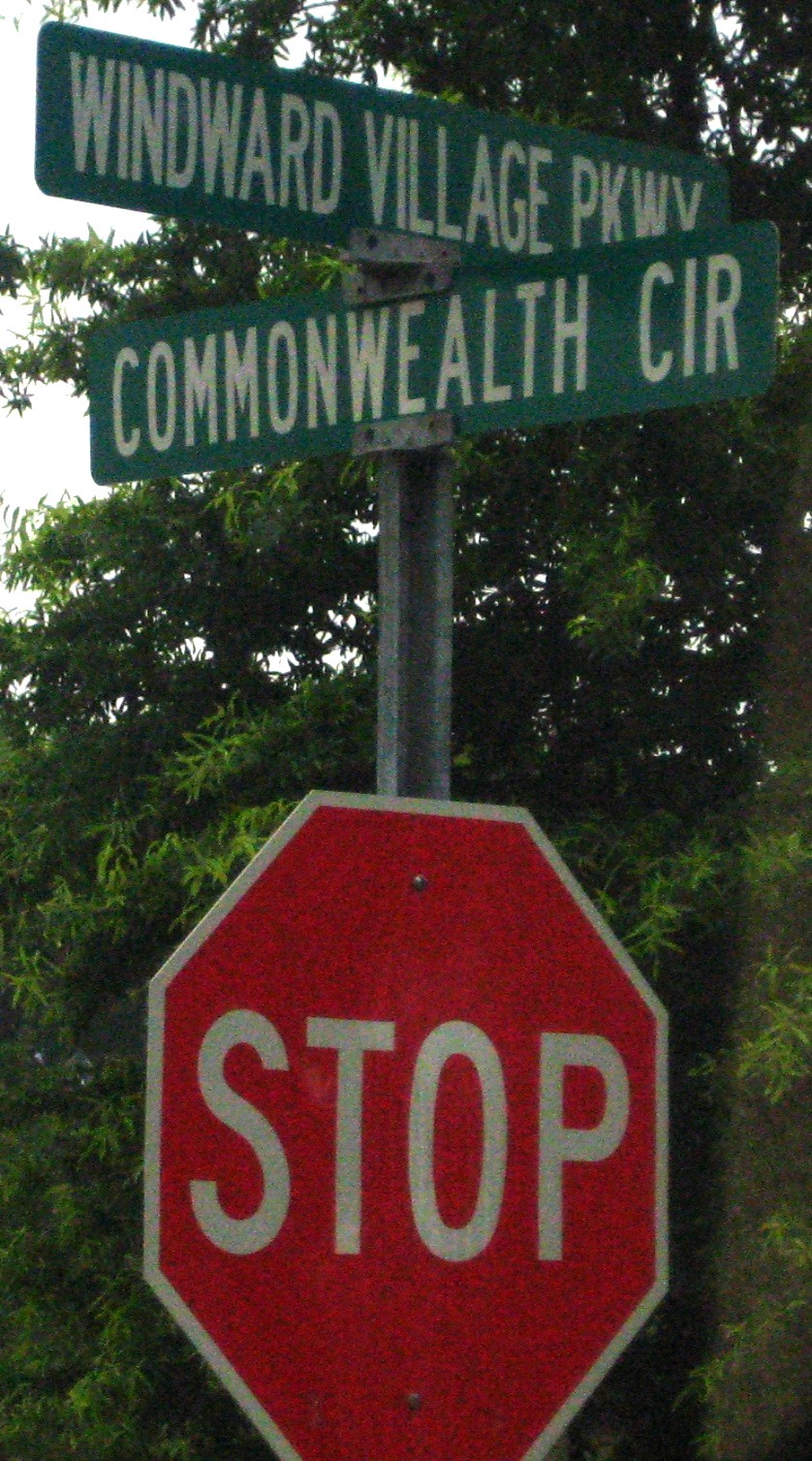The image is a detailed, daytime photograph featuring a metal pole that supports a series of signs. The sky is overcast, evident by the cloudy, sun-obscured backdrop. At the base of the metal pole, about nine feet tall, is a standard red stop sign with white lettering. Above it, there are two green street signs with white lettering. The top sign reads "Windward Village Parkway" and is oriented horizontally, while below it, a second sign reads "Commonwealth CIR" in a vertical orientation, giving a crisscross pattern. Surrounding the pole, there are vibrant green leaves from nearby trees, creating a lush, leafy background. The sky seen through the gaps in the foliage appears white due to the thick cloud cover.